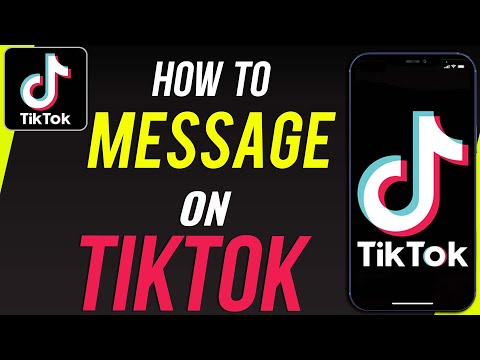A detailed and cleaned-up caption for the image could be:

"A smartphone displaying the TikTok app is shown in a screenshot. The TikTok logo, located in the upper left corner of the image, is also visible on the phone's screen. The screen features the instructional text 'How to message on TikTok,' with a black background. The text is color-coded: 'How to' appears in white, 'message' in yellow, 'on' in white, and 'TikTok' in red. The overall theme of the image is to guide users on messaging within the TikTok app."